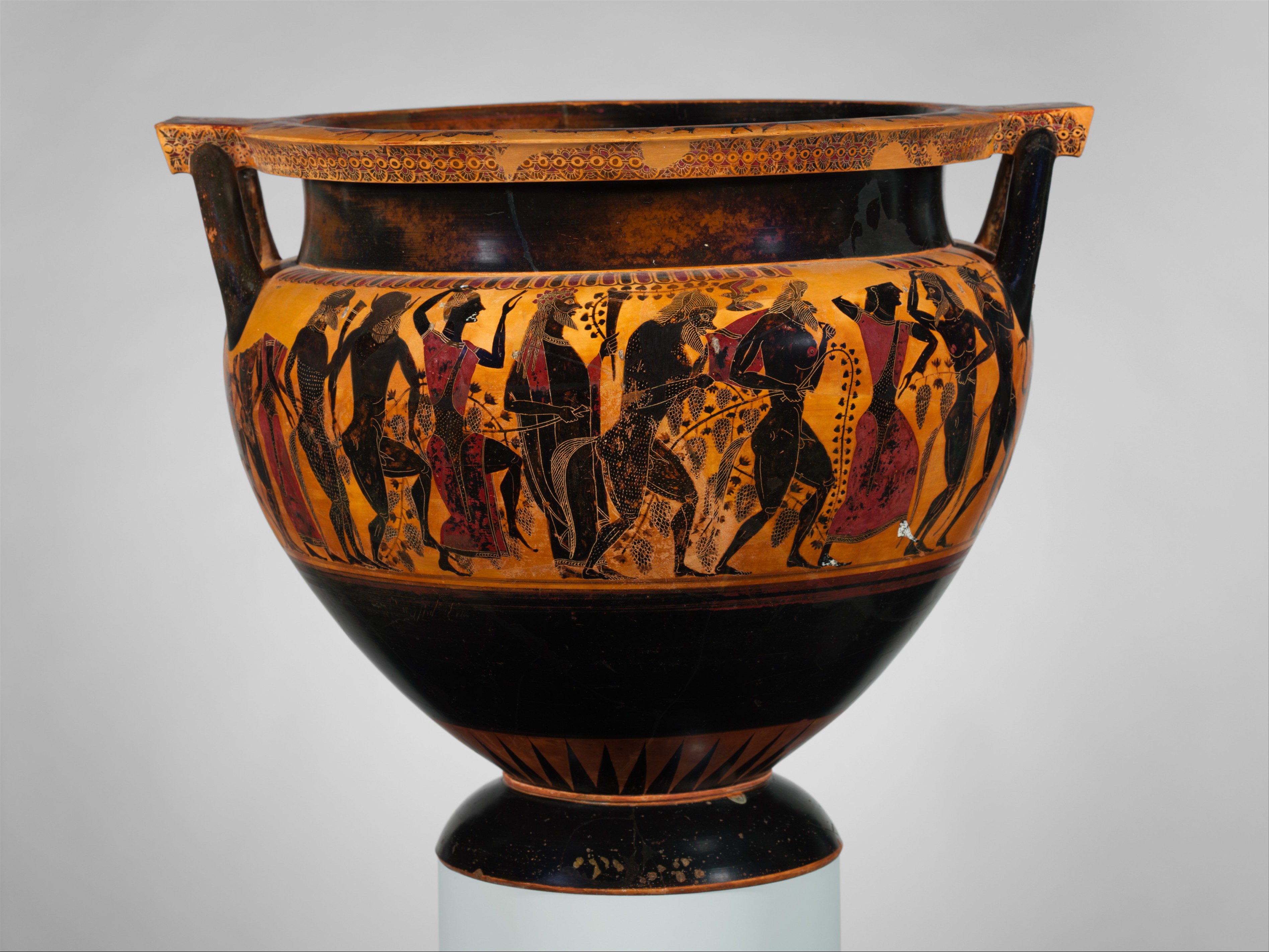This is a photograph of a Grecian urn, possibly an authentic antique or a high-quality reproduction, displayed against an all-white background. The urn is vaguely heart-shaped, broader at the top with a circular opening that matches its maximum width, suggesting it was designed to hold liquid. It rests on a circular brass base, which complements its predominantly brass appearance. The urn is beautifully adorned with a lighter colored band around its upper portion, featuring ornate illustrations of people in various poses. Notably, the design encircles the urn, depicting the god Pan playing his pipe, accompanied by dancers and musicians in a ceremonial parade. The background of the illustrated band is a yellowish-golden hue, which contrasts elegantly with the black trim that runs around both the base and the top edge of the urn. The urn has two discreet handles, adding to its functional yet aesthetic design. Repeating motifs of black and gold highlight the urn's edges and provide a sophisticated, decorative element to the overall piece, making it resemble a museum artifact.